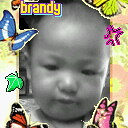This image is of a small digital card featuring a black and white photo of a young girl named Brandy, whose name is prominently displayed in yellow text with a purple outline at the top left of the card. The girl appears to be around two years old and possibly of Asian descent, with very little to no hair. She stands with a solemn expression, looking down at something off-frame, giving an impression of deep contemplation or curiosity.

The card is intricately decorated, with a vibrant and colorful border comprising computer-generated, pixelated images. Surrounding the photo are various elements: a blue butterfly, a green leaf, a red butterfly, and a pink butterfly on the right side. Additionally, there's a red leaf, a green leaf, a cat at the bottom right corner, and a pink symbol. Notably, there is also a purple adornment visible in her hair on the right side. Some of these elements, particularly the butterflies and leaves, are repeated in different colors, adding to the card's elaborate and whimsical design.